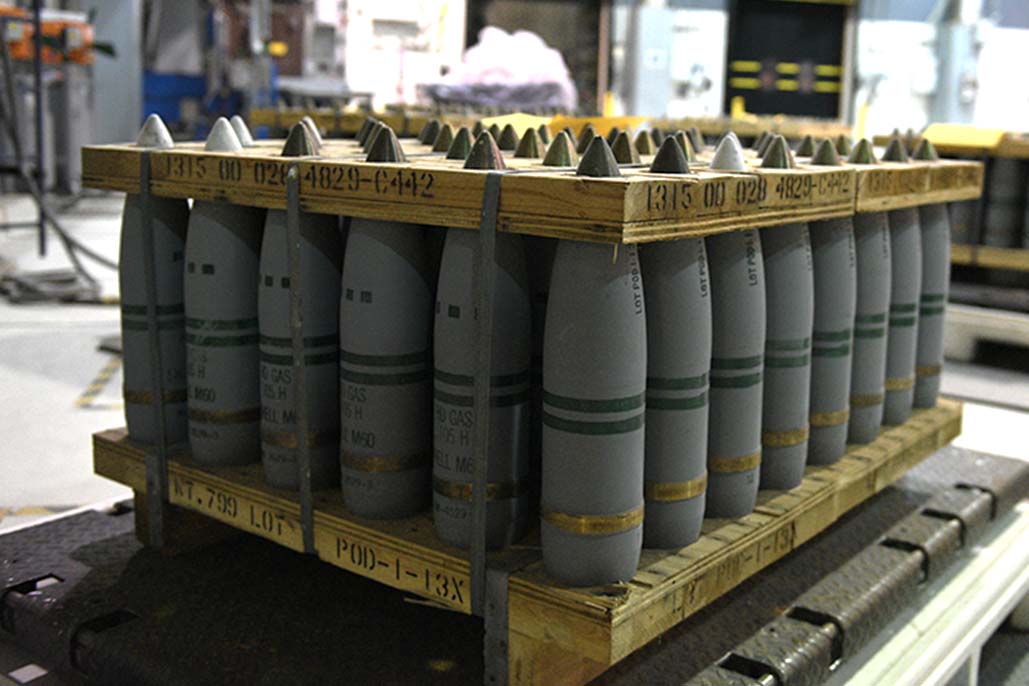The color photograph captures a detailed scene inside what appears to be a warehouse or a military area. Central to the image is a robust wooden crate, functioning as a pallet, which securely holds an orderly 6x8 grid of rockets or missiles. These projectiles, gray with black stripes, protrude through cut-out sections in the wooden top, allowing their tips to be visible. Metal straps efficiently secure the wooden pieces together, ensuring the stability of the load, which rests on a black plastic mat. Specific markings are visible on the crate and the missiles; the side of the bottom crate is labeled "799 lot POD-1-13X," while the top edge of the crate and the right side of the missile enclosure bear the number "1315 00 028 4829 C442". Despite some illegible writing on the missiles, the overall setup is clearly captured in the well-lit, spacious setting, which lacks visible personnel or animals. The backdrop of the room remains out of focus, adding an air of mystery to the precise and orderly arrangement in the foreground.